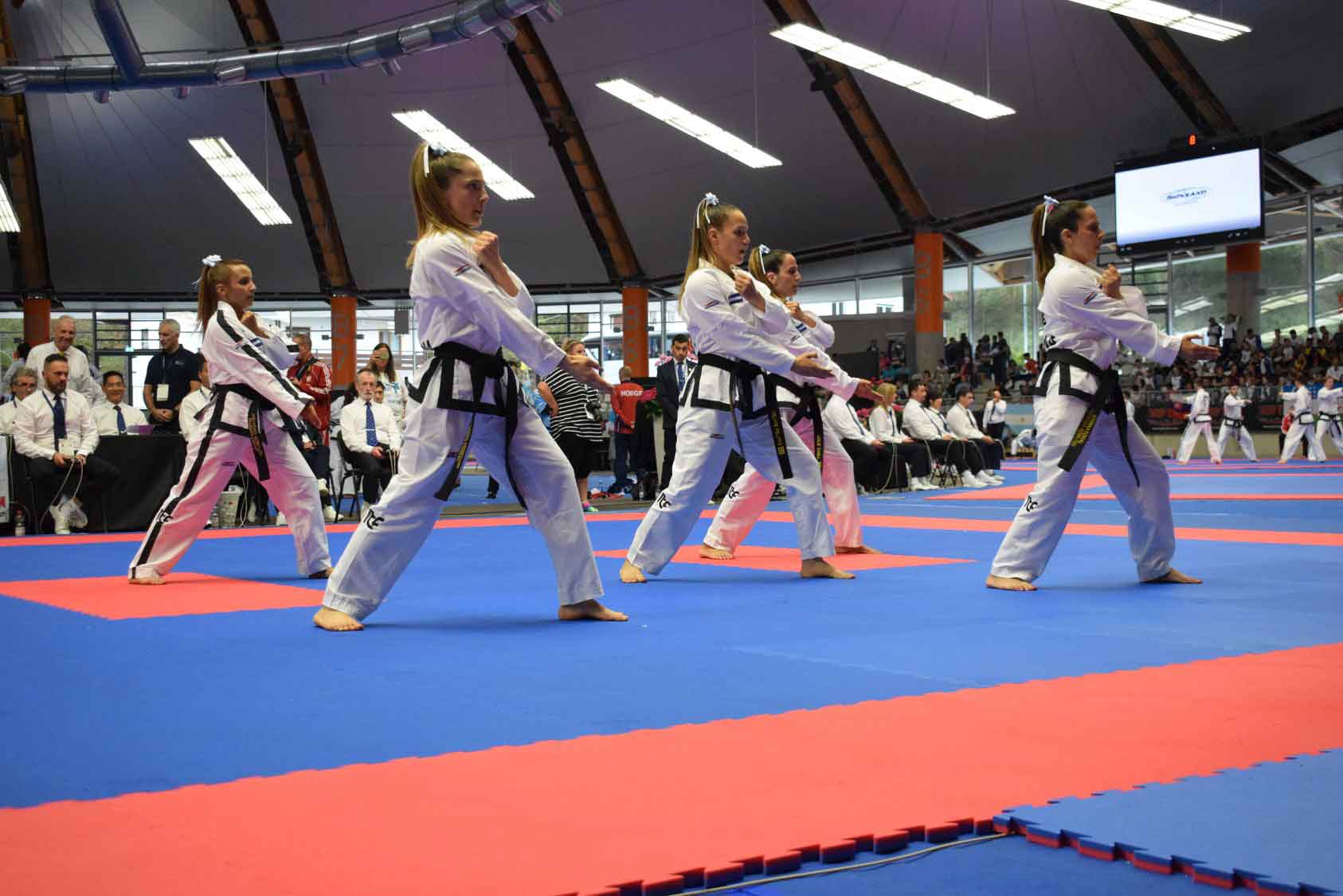The photograph captures a dynamic scene from a judo or karate class featuring five young women in traditional martial arts uniforms. They are arranged in a formation with two on the left, one in the middle, and two on the right, performing an exercise with their right arms extended diagonally downwards, fingers pointed out. Each woman is barefoot, wearing a uniform adorned with black and white belts, and some have black trim on their outfits. The women also have white ribbons or similar adornments in their hair. The action takes place on a red and blue mat, which serves as their dojo floor. 

In the background, a diverse audience is visible, comprising seated and standing spectators, as well as other individuals in martial arts outfits walking across the space from the right. The venue is brightly lit, revealing a ceiling characterized by a white tile design and metal casings, with windows integrated into the structure. A large monitor is positioned on the right side of the image, although its display is blurry and difficult to decipher. The setting resembles an exhibition space with a distinctive architectural style featuring columns and large glass windows, suggesting an expansive and open atmosphere conducive to public viewing.